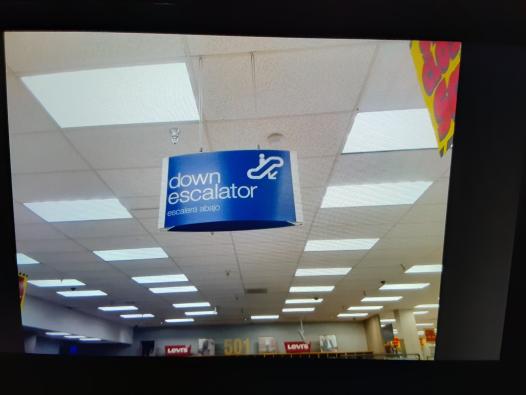This photograph captures the interior of a department store, primarily focusing on a blue sign hanging from a white drop panel ceiling. The ceiling features a repeating pattern of square lights and fire sprinklers. Centrally displayed, the sign reads "Down Escalator" in bold white text, accompanied by a pictogram of a stick figure descending an escalator, and includes a Spanish translation below. In the distant background, merchandise and signage are just barely visible, including two red Levi's logos and the number "501," indicative of a section selling jeans. The image also includes a yellow sign with red lettering in the upper right corner, partially cut off, adding to the busy backdrop of the store.